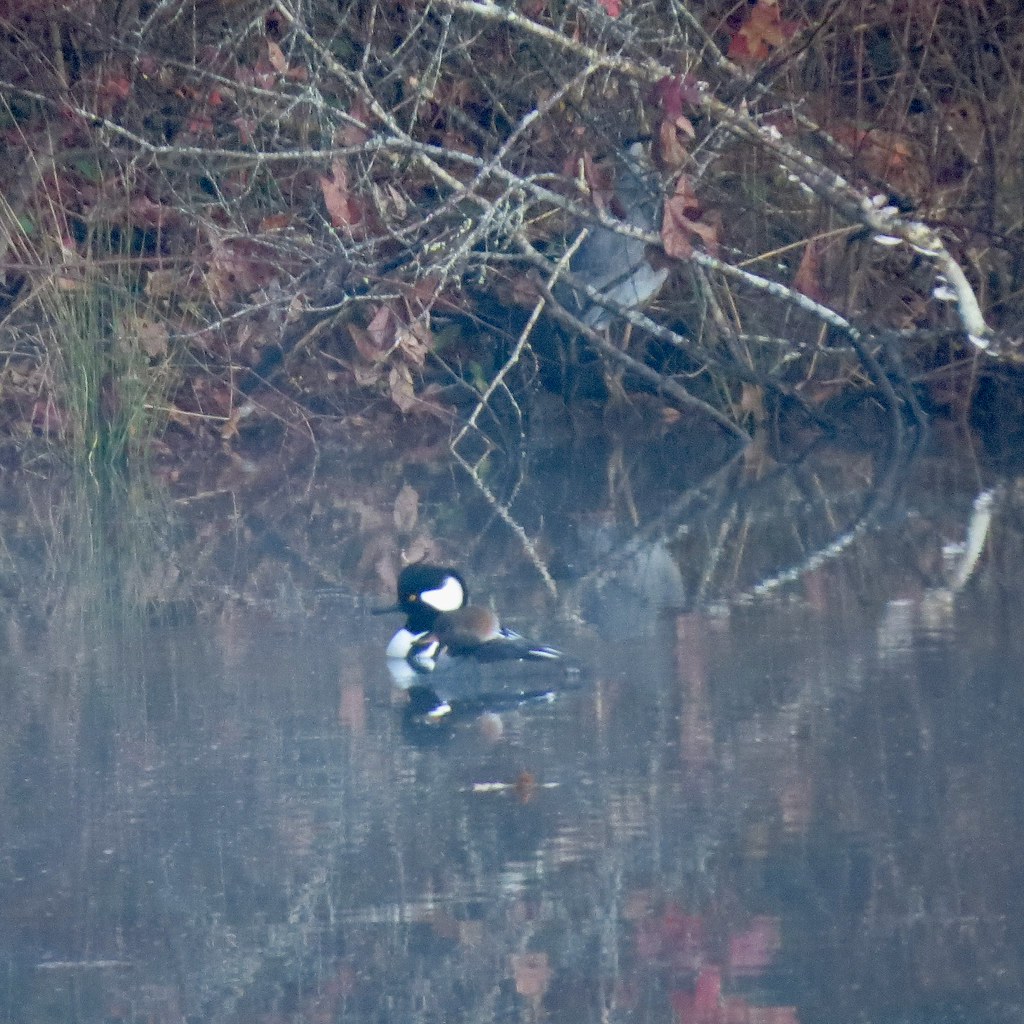In the image, a striking bird swims gracefully in a murky pond, surrounded by the reflections of a dense background of twigs, fallen plants, and dried leaves. The bird, the central focus, is slightly off-centered. It features a distinctive black head with a small black beak and an orange eye. A half-moon shape of white adorns the very right side of its head, blending seamlessly into its white chest. Its feathers transition from a blackish hue to gray and brown on its back, with its tail feathers ending in black, with tips of white. The tranquil scene is further enriched by the mirrored images of the bird and the surrounding branches of brown and white, along with a hint of greenery on the right, all captured in the serene waters of the small pond.